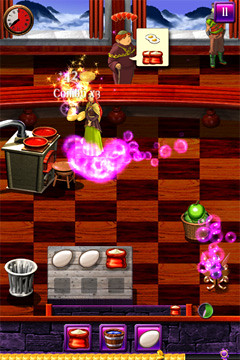The image is a detailed screenshot from a cooking-themed video game. The scene is set inside a cozy kitchen with a predominantly orange and red checkerboard-patterned floor. Towards the background, two large windows offer a picturesque view of snow-capped mountains. Between the windows stands a character resembling a monk, dressed in a brown robe with reddish-orange hair, surrounded by hearts and a speech bubble indicating ingredients. The speech bubble displays two eggs and what might be mushrooms. In front of this character, there's a stove with two burners, each hosting a pot, and a wooden chair positioned nearby. A female character wearing a green dress over a brown shirt, with reddish-orange hair, is seen at the stove, which appears to be grey with red interiors. A pink cloud-like aura surrounds her feet, suggesting some special activity or power. At the bottom of the screen lies a table featuring two eggs and a red bag, possibly containing flour, alongside a trash can and other cooking elements.